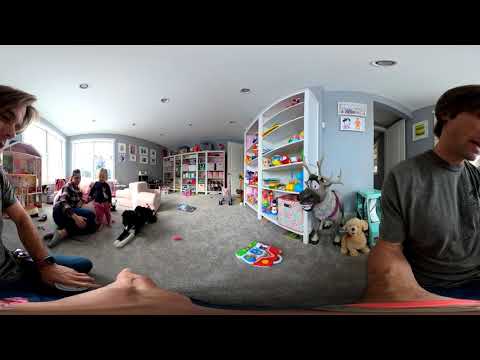In the image, we see a detailed and expansive 360-degree panorama of a playroom. The panoramic effect causes the scene to appear somewhat skewed, giving it a fish-eye lens feel. To the left, a man is holding up a camera, with his arm extended towards the lens, and his face visible from the front. As the panorama unfolds, his body wraps around the image, with his right side showing the back of his head and his torso clad in a gray t-shirt and jeans.

The room itself is large and appears to be a cozy playroom, featuring gray carpeting and a myriad of colorful toys scattered around. Prominent shelves and bookshelves, flush with vibrant toys in shades of red, yellow, blue, and pink, line the background. On the floor, a small stuffed goat and puppy can be seen, adding to the playful atmosphere.

Towards the left, near some floor-to-ceiling windows adorned with pictures, a woman in a striped top and jeans sits beside a toddler dressed in a dark top and pink pants. Nearby, a stuffed dog and a pink toy house contribute to the lively clutter.

Overall, the room exudes a cheerful and family-oriented environment, with an abundance of playthings and a clear sense of joyful disarray perfect for kids.